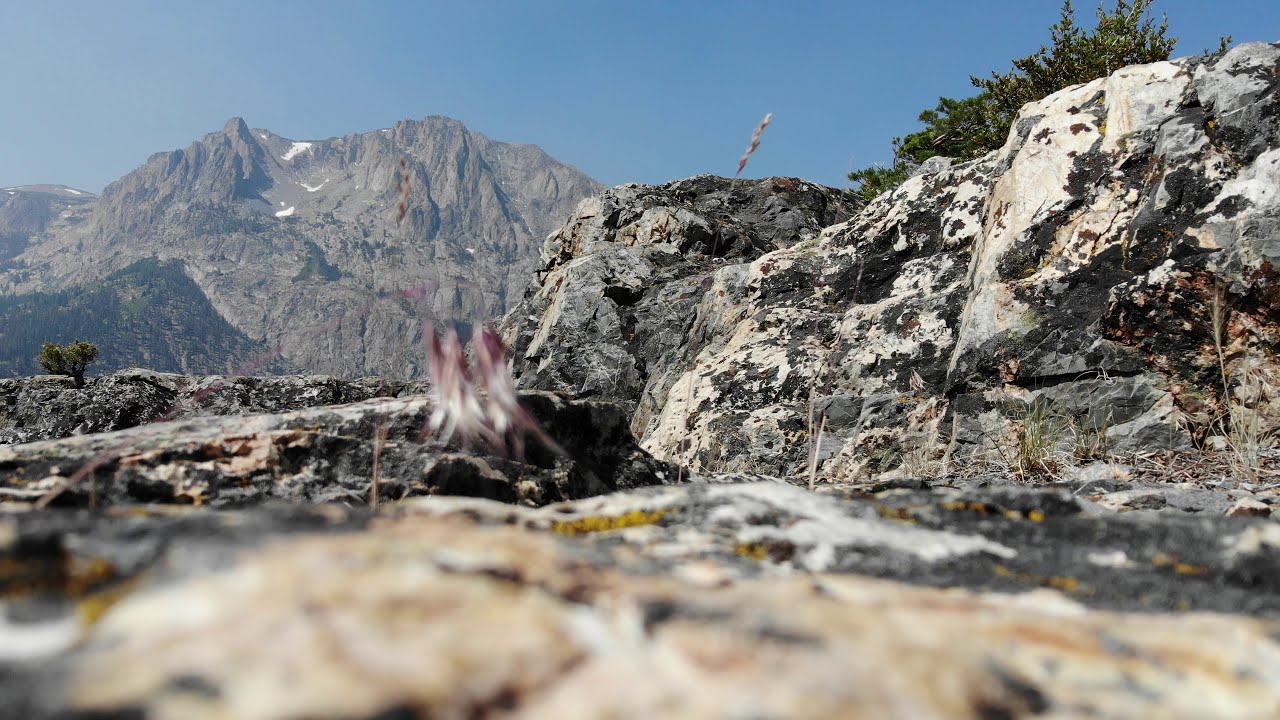This image portrays a rugged outdoor landscape dominated by a distant, rocky mountain with patches of snow near its summit. The mountain, steep and grey, serves as the primary focal point, while a hillside dotted with pine trees forms its base. The photograph was taken during the daytime, under a mostly clear blue sky which fills the upper portion of the frame. In the immediate foreground, there's a vaguely out-of-focus scene of rocky gravel with scattered plants, including a distinctive yellow spot and some white and pink elements that might be weeds or flowers. Off to the right, a rocky hill is adorned with green bushes. Interestingly, a long, thin man-made object resembling a spear, detailed with feather-like adornments, is embedded in the rock. The overall color palette includes shades of green, white, grey, blue, and hints of pink. The perspective suggests the camera was positioned closely to the ground, emphasizing the near details of rocks and sticks before leading the viewer’s eye towards the distant mountainous backdrop.